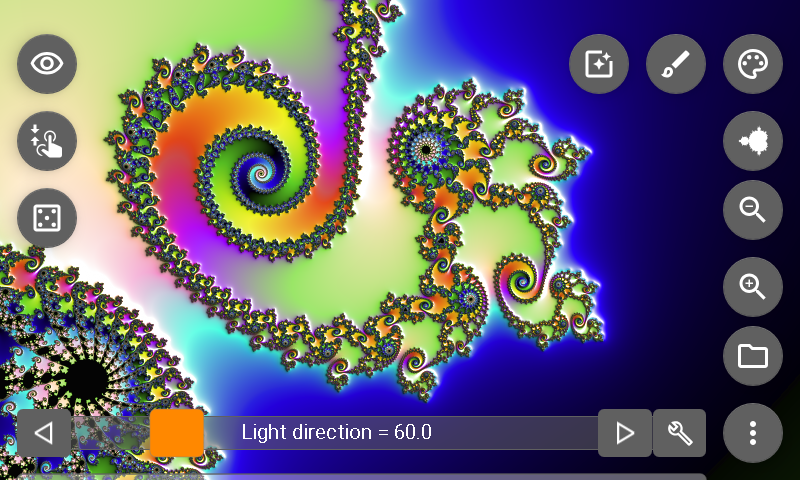The image is a detailed screenshot of a digital art application, showcasing a vibrant piece of artwork in progress. The background of the artwork is a deep, dark blue, overlaid with an intricate paisley pattern characterized by multicolored swirls in greens, pinks, yellows, oranges, and purples. The swirls converge to points, creating a dynamic yet harmonious design.

The main focus of the artwork resembles a curlicue chain that wraps around a central shape, akin to an eyeball with a black center surrounded by jewel-like elements in pink and blue hues. The entire composition is vibrant, with colors melding together to create a fluid rainbow effect.

Around the border of the artwork, gray circles with white icons denote various tools available in the application. On the right side, there's a vertical row of six icons including a paint palette for color selection, magnifying glasses for zooming in and out, among others. The bottom part of the interface features a bar to adjust light direction with a value of 60.0, flanked by arrows pointing left and right and a small gold star icon.

In the upper left corner, additional gray circles contain icons such as an eye for visibility, a pointing finger, and a square with five dots, suggesting interactive tools for enhancing or modifying the artwork. The interface design reinforces that this is a sophisticated digital art application, offering various controls to aid in the creative process.